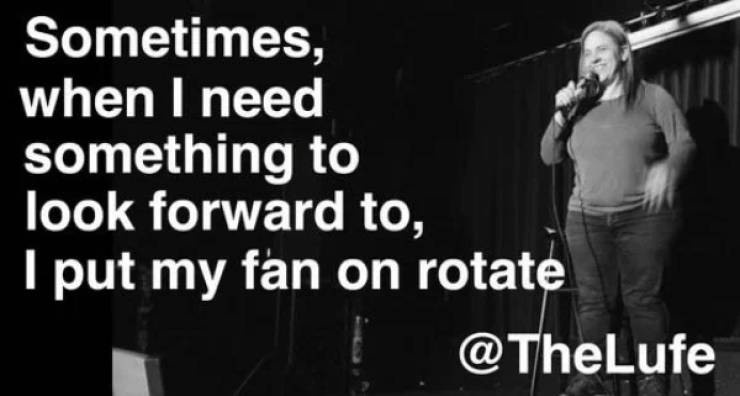In this black and white photograph, a woman stands on stage at a comedy club, positioned on the right side of the image. She's wearing a long-sleeve shirt and jeans, holding a microphone in her right hand up to her mouth, while her left hand is slightly blurred, indicating movement. Her smile suggests that she is likely delivering a punchline to an unseen audience. Behind her, a black curtain provides a stark yet complementary backdrop. On the left side of the image, white Arial bold text, cascading from the top left, reads, "Sometimes when I need something to look forward to, I put my fan on rotate." In the bottom right corner, the text "@TheLoof" indicates the name of the club.